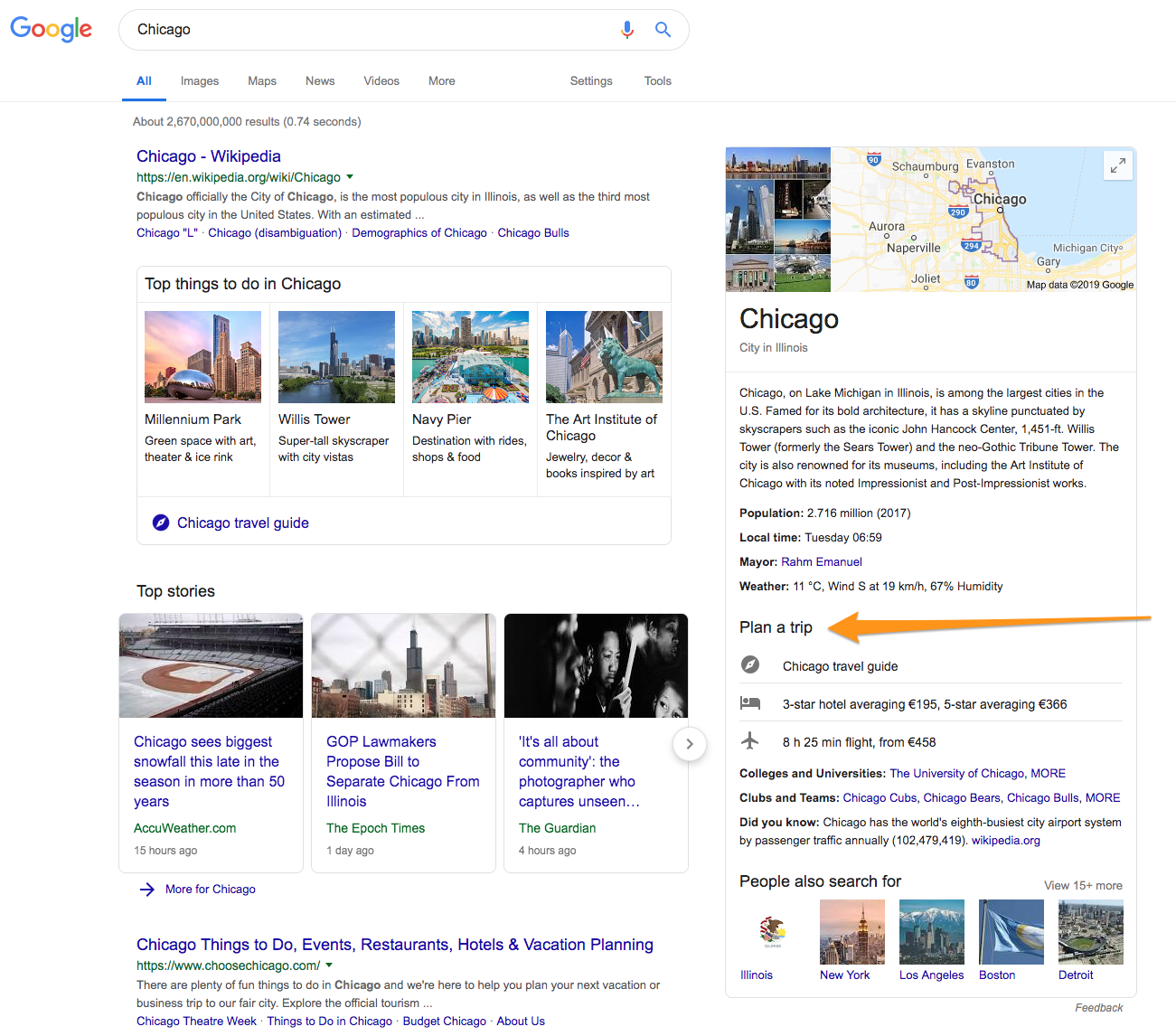The image depicts a screenshot of a Google search page with the query "Chicago." At the top, a blue line highlights the "All" tab, indicating that all types of content are shown, which could be switched to view images, maps, news, videos, and more, or adjusted using settings and tools.

On the left side of the screen, the first result is a link to the "Chicago - Wikipedia" page, providing comprehensive information about the city. Below this, a list appears under "Top things to do in Chicago," featuring key attractions: Millennium Park, Willis Tower, Navy Pier, and the Art Institute of Chicago.

Further down, the "Top stories" section is shown with three headlines: "Chicago sees biggest snowfall this late in the season in more than 50 years," "GOP lawmakers propose bill to separate Chicago from Illinois," and "It's all about community: the photographer who captures unseen..."

Along the right side of the page, a map of Chicago is displayed, pinpointing the city's location. An orange arrow extends across the page next to a "Plan a trip" link, encouraging users to explore travel options. The section "People also search for" is also visible, suggesting additional related queries.

Overall, the image captures a comprehensive and interactive Google search results page, offering a variety of resources and information about Chicago.